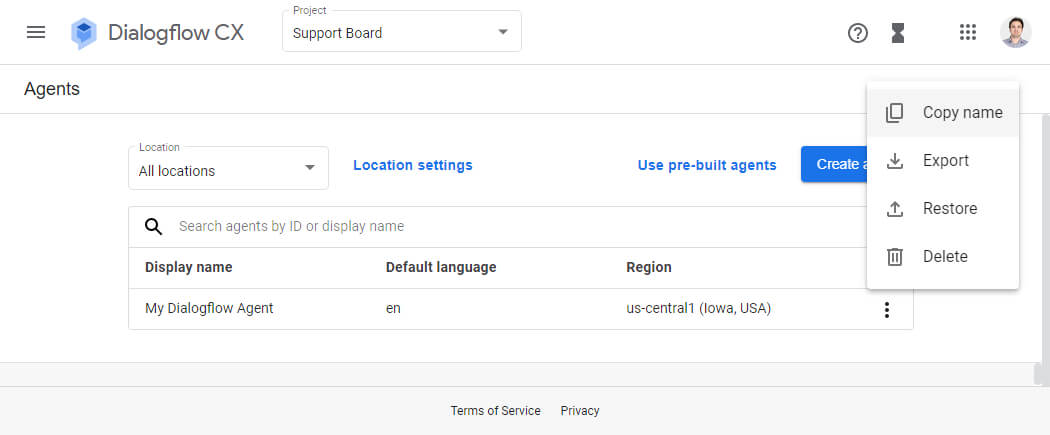This image is a detailed screenshot of a website interface set against a solid white background. At the upper left corner of the header, there is a menu icon. Adjacent to it, a blue cube logo is prominently displayed. Next to the logo, in large gray text, the words "Dialogflow CX" are clearly visible. Moving further to the right, there is a white box featuring a pull-down menu, labeled "Project Support Board." 

In the upper right corner of the header, another menu icon is present, along with a circular image of a man's face, indicating the user's profile.

Below the header, on the left side, the word "Agents" appears in gray text against the white background. Beneath this, a location button with a pull-down menu is visible, labeled "All Locations Inside." To its right, in blue text, are the words "Location Settings," and further to the right, also in blue text, it reads "Use Pre-Built Agents." Below these options, there is a conspicuous blue action button labeled "Create."

Further down the page, bold black text spans from left to right, listing "Display Name," "Default Language," and "Region." This area seems to be involved in setting or viewing the characteristics and configurations of various projects or agents on the website.